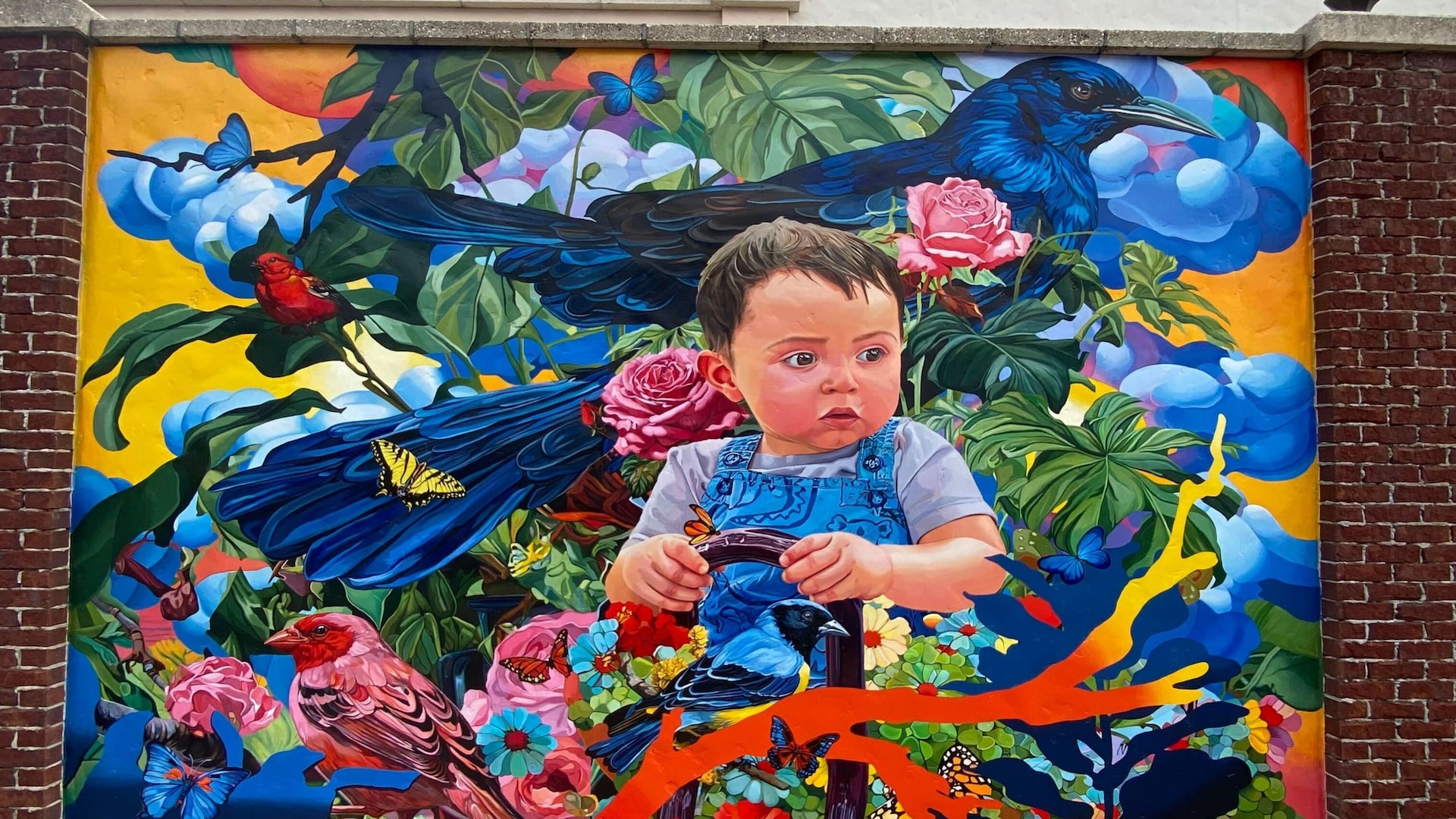This vibrant mural, painted on an outdoor brick wall, depicts a young Caucasian boy, approximately one to two years old, with light brown hair. The child is at the center of the mural, seated and wearing blue overalls over a light blue short-sleeve t-shirt. He appears to be holding a cane or perhaps a steering wheel, looking slightly to his left. The bright and complex background features a striking combination of pastel hues and natural elements: a warm yellow and orange sky transitions to a scene of clouds represented by blue bubbles, amid a plethora of greenery and multicolored flowers, primarily in blues and pinks.

Surrounding the child are several birds of varying colors. Directly behind him is an enlarged portrait of a black crow. To the right, perched on a branch, is a vibrant red bird, and below the crow’s tail, a yellow butterfly rests. Additionally, another bird, colored blue with black and yellow accents on its breast, sits in front of the boy. Overall, this mural with its detailed flora, winged creatures, and playful depiction of the child, brings life and color to the once plain brick wall. Noticeably, there are no signs or writings within the image.